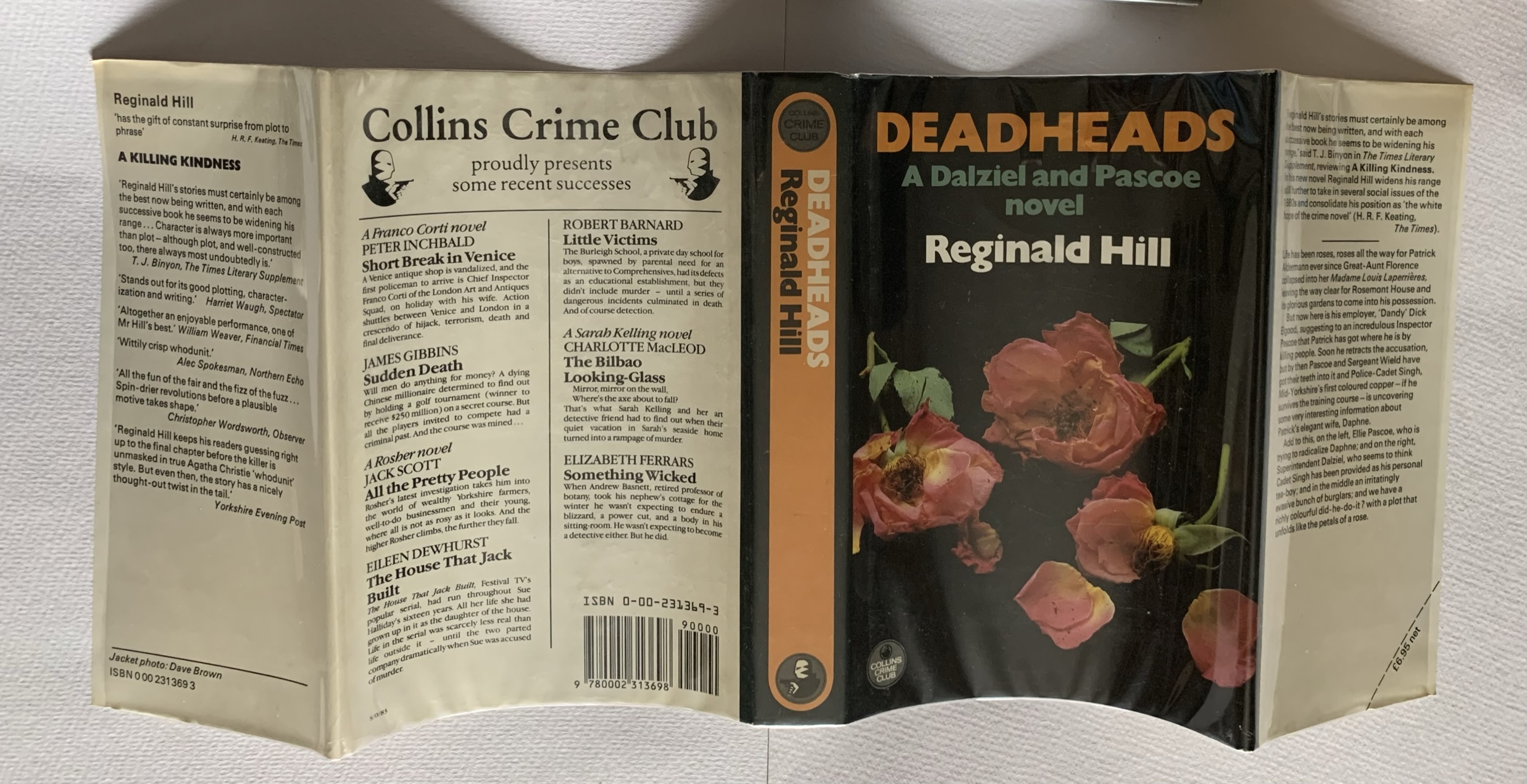This image showcases the front and back covers of a well-worn book titled "Deadheads," a Dalziel and Pascoe novel by Reginald Hill. The book cover exhibits signs of age, with yellowed pages and a slightly beat-up condition. Prominent colors on the front cover include shades of orange, black, white, and a sage-like green. The cover art features wilted roses against a dark black background, symbolizing the "dead heads" referenced in the title. 

The back of the book indicates its affiliation with the Collins Crime Club and highlights some recent successes by other well-known authors such as Richard Bernard's "Little Victims," Elizabeth Ferris's "Something Wicked," Jack Scott's "All the Pretty People," and James Gibbons's "Sudden Death." Inside the book, on the second page, there is a summary of the novel. The spine of the book, also visible in the image, adds to the detailed exploration of its well-loved state.